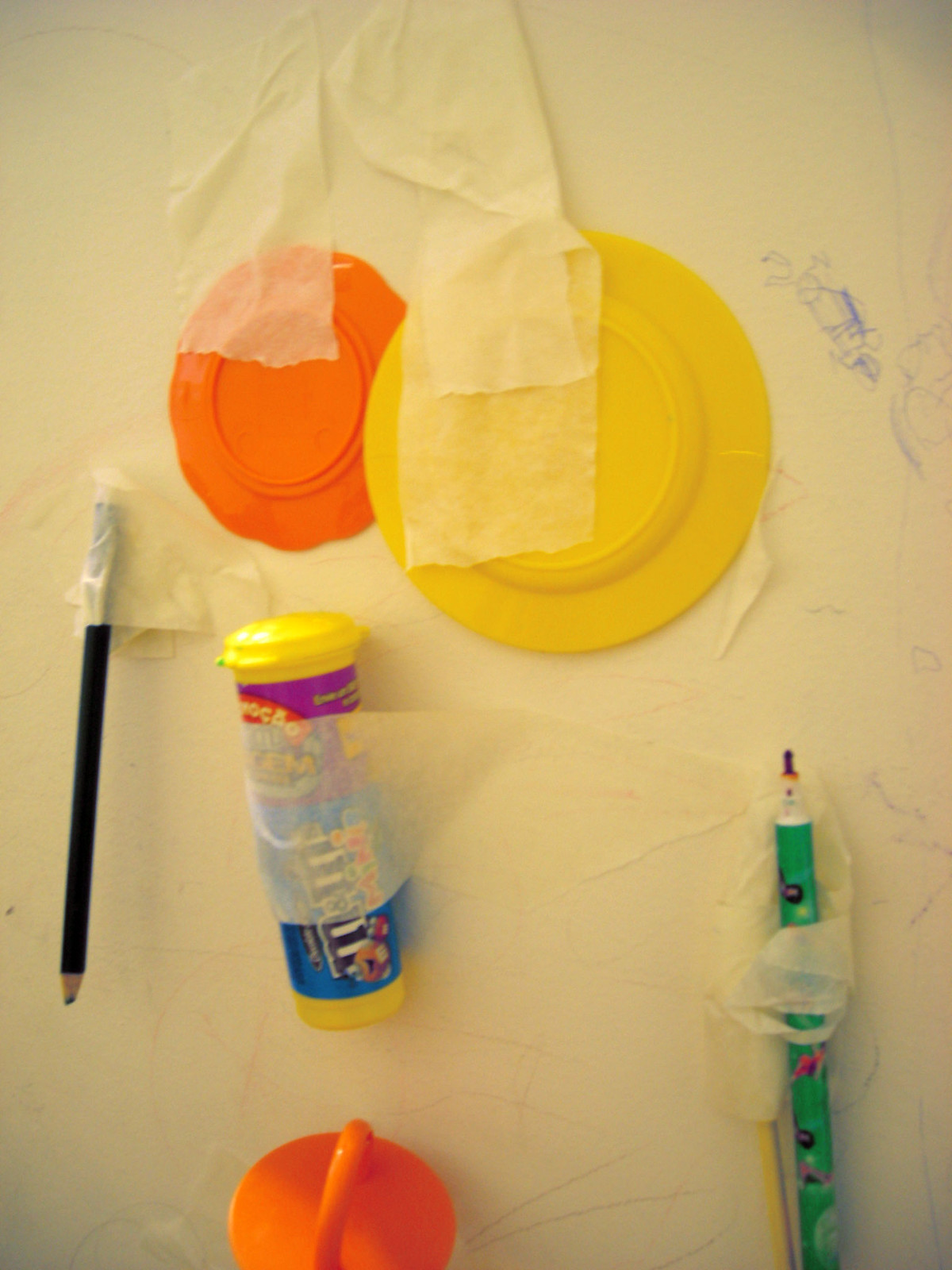The image showcases a whimsical art project, likely created by a child, displayed against a plain white wall. On the right-hand side, thin scribble marks in blue, suggestive of a blue ballpoint pen, are scattered haphazardly. Various objects are affixed to the wall using white tape, adding a textured and three-dimensional quality to the artwork.

Positioned towards the upper-left area of the composition is an upside-down orange plate, slightly overlapping with a larger yellow plate nearby. Both plates are securely taped from the top edges. Below the orange plate, slightly to the left, is a black pencil, also taped at the top. Adjacent to the pencil is a tube of mini M&Ms, distinguished by its yellow cap and body, featuring a label transitioning from purple to blue. The familiar brown M&Ms logo and anthropomorphic M&M characters, reminiscent of those in commercials, adorn the label.

Beneath the M&Ms tube is an orange object resembling a disc with a handle protruding from its center, though its method of attachment remains unclear. To the far right of the composition, a green felt pen, possibly felt-tipped, is taped to the wall, with the tape artistically woven around it. This eclectic assortment of everyday items, combined with the spontaneous blue scribbles, creates a playful and imaginative display.